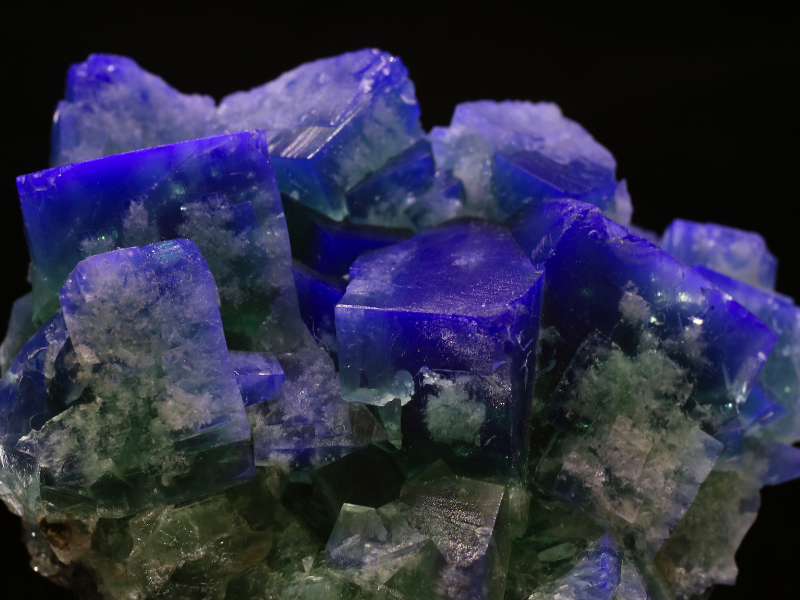This image showcases a professional, close-up photograph of a mineral cluster set against a black background. Dominating the shot are deeply vivid blue to violet crystals with distinct, straight lines, forming what look like large, squarish shapes. These crystals, possibly magnified, exhibit a vaguely translucent quality, hinting at their ability to allow some light to pass through. Appearing almost fluorescent, these deep-hued crystals are visually striking. Nestled among them are smaller, greenish jade-colored crystals—particularly towards the bottom and sides—adding to the intricate beauty of the cluster. The greenish crystals, moderately see-through and non-fluorescent, contribute to the overall crystalline quality of this natural formation, reminiscent of a jumble of dice with a mix of vivid blues and interspersed greens. The lack of any object for scale in the image leaves the exact size of the crystals open to interpretation, yet the photograph captures their mesmerizing, crystalline structure in remarkable detail.